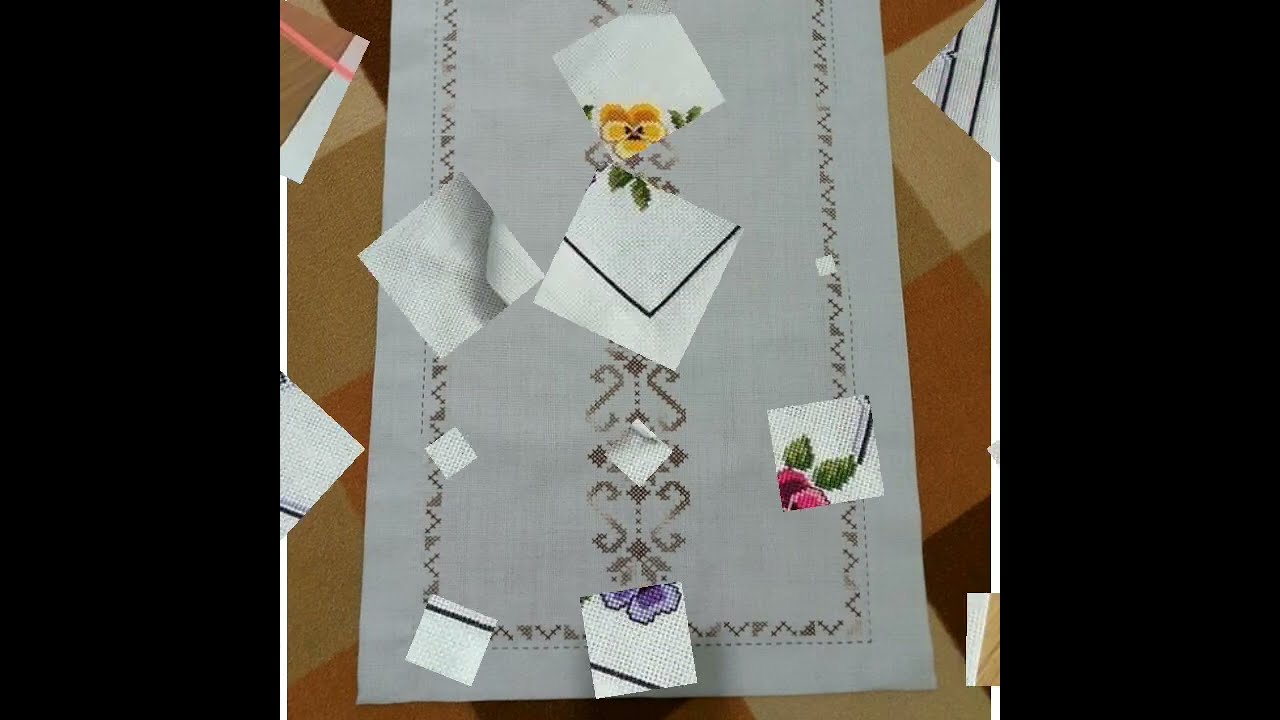The image depicts a light green, rectangular piece of paper set against a complex, multicolored surface featuring dark yellow, cream, and light green squares. This background resembles an intricate cross-stitch table runner, extending beyond the frame with a mix of colors including tan, brown, and gray, and sprinkled with various geometric shapes like triangles and other polygons. Additionally, it has two vertical black strips on either side. The central rectangular paper boasts detailed designs both on the edges and in the middle. Scattered atop this paper are numerous square cuttings, each showcasing different cross-stitched floral designs — including yellow, pink, and blue flowers — positioned randomly. Some of these cuttings also spill over onto the background surface, enhancing the layered, collage-like aesthetic of the image.